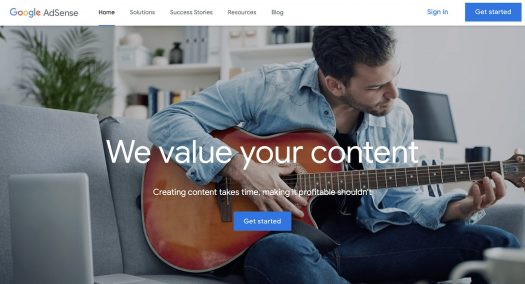The image, sourced from a webpage, prominently features the Google AdSense home interface. At the top, against a white background, are navigation links labeled "Home," "Solutions," "Success Stories," "Resources," and "Blog." To the right, there are two interactive options: "Sign In," displayed in blue text, and "Get Started," presented within a blue box with white text.

Below this header, a man sits on a bluish-gray couch, focused intently on strumming an acoustic guitar. He dons a stonewashed denim shirt with rolled-up sleeves and a turned-down collar. Above him, a banner reads, "Creating content takes time, making it profitable shouldn't." Near the bottom of the image, there's another blue "Get Started" button, inviting further interaction. The overall composition captures the convergence of creativity and monetization through Google's platform.